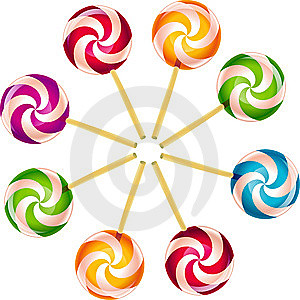In this vividly detailed artistic pop art image, eight lollipops with swirled patterns of various colors—green and white, purple and white, red and white, orange and white, yellow and white, darker green and white, blue and white, and another red and white—are meticulously arranged in a circular formation. Each lollipop is depicted with a stick that converges towards the center but doesn't quite touch, forming a geometrically pleasing pinwheel effect. The lollipops are rendered with a three-dimensional quality, their sticks resting on the dotted edge of a small white circle. The background features a subtle, pale gray swirl that emanates from the central white circle and spirals outward, adding depth and motion to the composition.